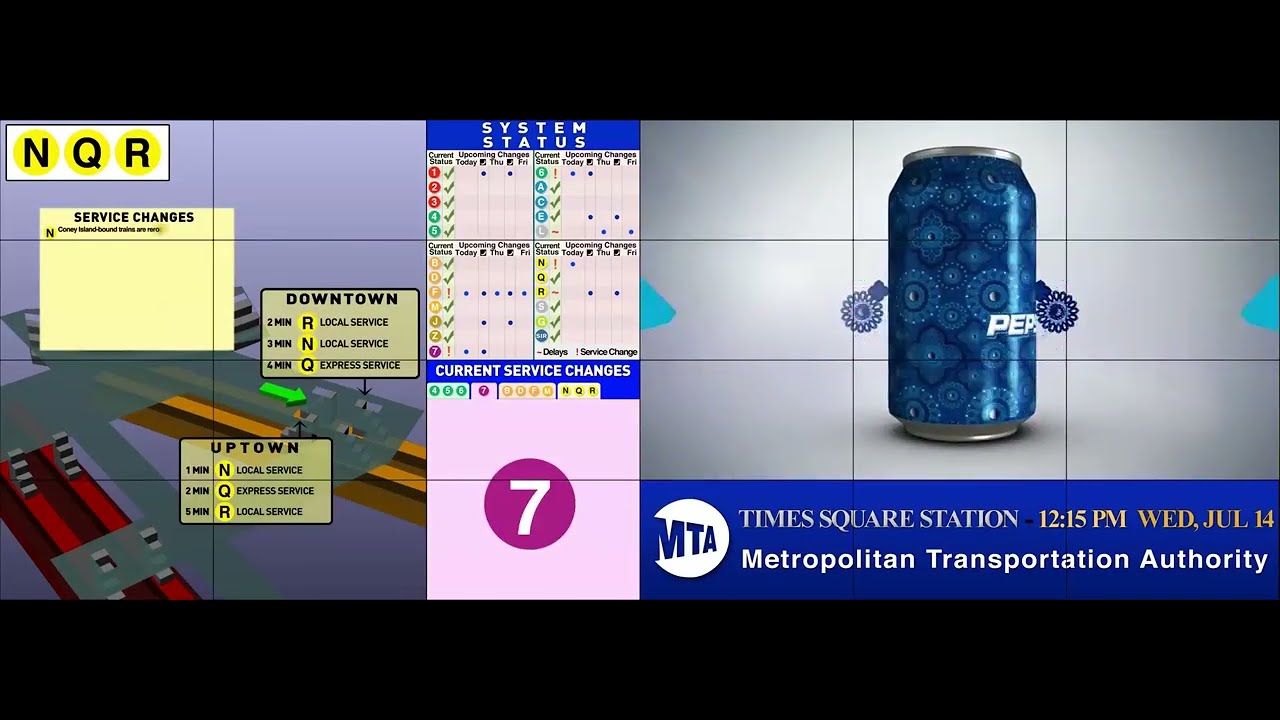This horizontal rectangular image, bordered by thick black bars at the top and bottom, combines three distinct sections. On the right side, there's an eye-catching, 3D-styled image of a Pepsi can, adorned with bubbles and geometric shapes giving the illusion of the can floating. The logo, predominantly blue with red and white, is surrounded by concentric circles in alternating blue and white, resembling targets or poker chips. Below the can, a blue box displays the text "Times Square Station, 12:15 PM, Wednesday, July 14th" followed by "Metropolitan Transportation Authority" and an MTA logo to the left.

The central part of the image features a focused segment on transportation updates. At the top, it says "System Status" in white letters on a blue background, and beneath it, "Current Service Changes" is highlighted. Various subway lines are listed, including the 1, 2, 3, 4, 5, 6, A, C, E, L, B, D, F, M, J, Z, 7, N, Q, and R trains.

On the left-hand side, a vertical rectangular section mimics a subway map. In the upper left corner, a white background with a black-bordered rectangle displays "NQR" in black letters within a yellow circle. Below are three boxes labeled "Service Changes," "Downtown," and "Uptown," detailing specific service updates. This part appears as a simplified representation of a typical MTA status board.